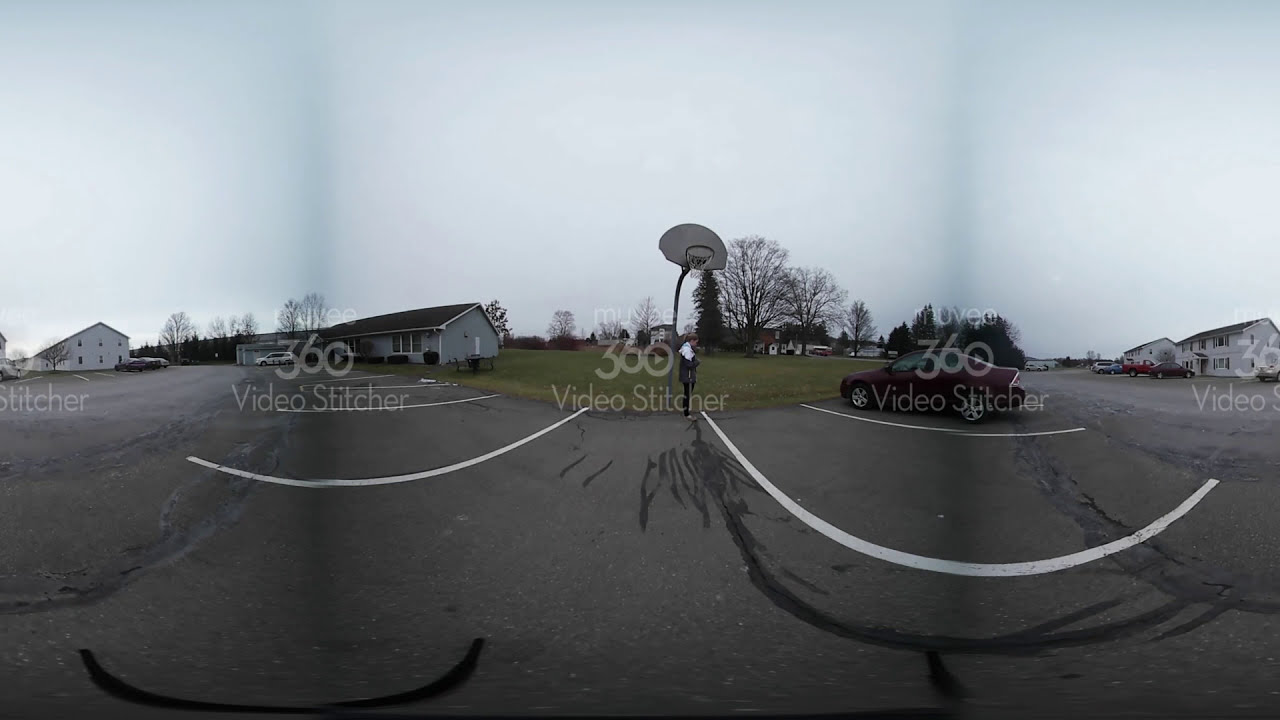The image depicts a suburban neighborhood under an overcast sky, with a prominent "360 video stitcher" watermark repeated multiple times across the scene. The central focus is a large asphalt parking lot with spacious parking spaces, bordered on the right by an apartment building and on the left by several light gray houses with gray roofs. A red car is parked in the lot, and a basketball hoop stands in the middle, near a large grassy area where a person is visible. The sky appears gray and tumultuous, with dark blue formations reminiscent of tornado clouds.